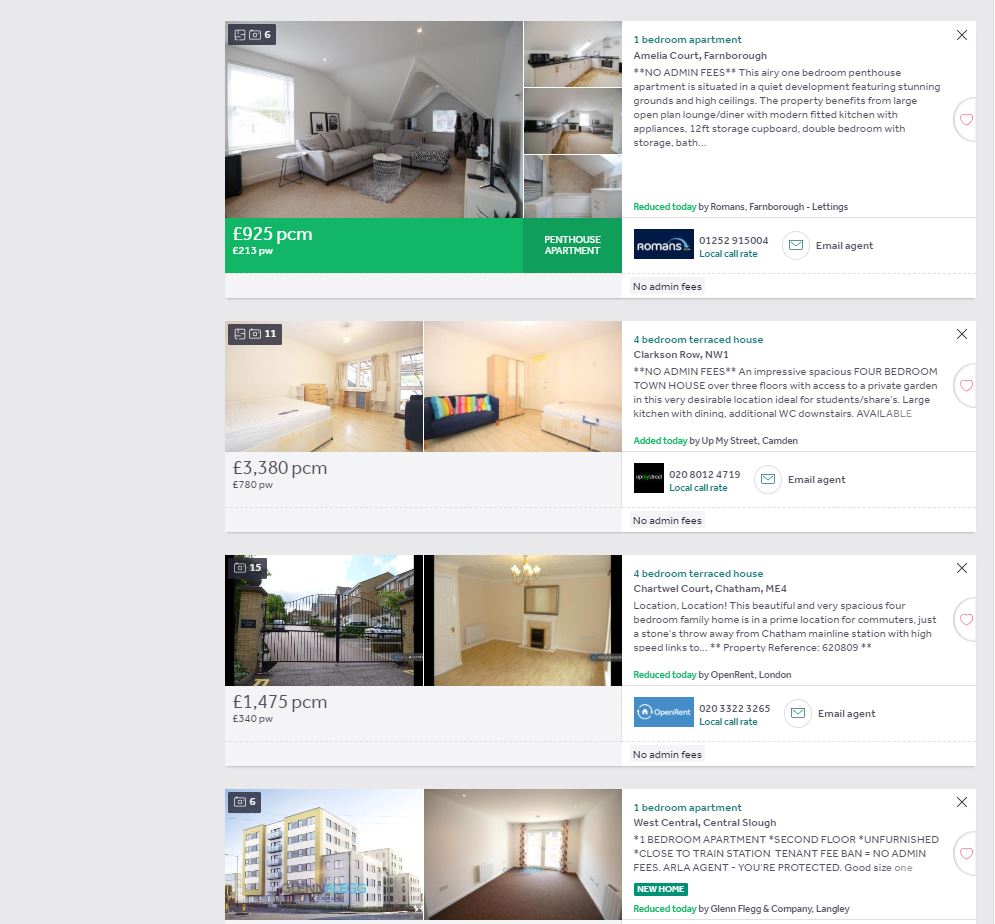The screenshot showcases a desktop version of a UK-based housing website, designed for browsing rental flats and houses. The image prominently displays three property listings with detailed rent prices and descriptions:

1. A one-bedroom apartment listed for £925 per calendar month (PCM).
2. A four-bedroom terraced house priced at £3,380 PCM.
3. Another four-bedroom terraced house available for £1,475 PCM.

A fourth listing, partially visible due to the screenshot's cut-off, appears to feature a three-bedroom apartment, although its rental price is obscured.

Each listing includes contact options such as phone numbers and email links to connect with the respective agents. Additionally, the website provides multiple images for each property, offering a visual tour of the rooms and amenities.